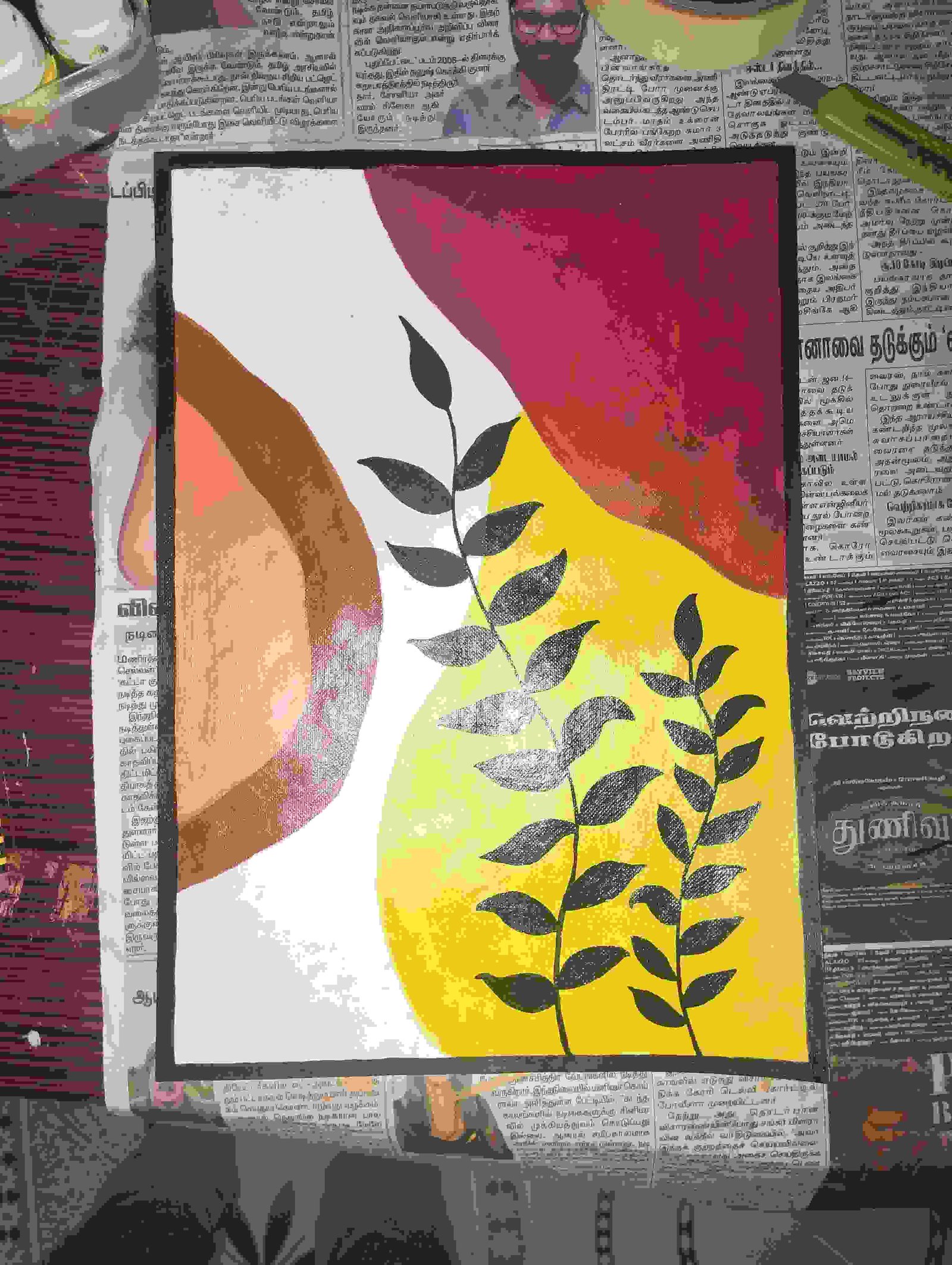This image features a detailed multimedia artwork with a modern aesthetic. The backdrop consists of newspaper clippings with a variety of articles, including one prominently displaying the face and shoulders of a dark-skinned man with glasses and a black beard. Surrounding this portrait are various sections of printed text. Along the right-hand side, set against the newspaper, is a green X-Acto knife with its blade slightly extended.

Central to the piece is a painting that appears to be set atop the newspaper clippings, giving the impression that the art is in the midst of being created. This painting includes two stylized plants with black leaves and stems, framed within a painted black rectangle. These plants rise in front of a yellow shape resembling a pear, overlaid with splotches of red, magenta, and orange. To the left of this central image is a brown semicircular shape with a thick border, housing hues of peach, tan, and darker taupe. The background of the painted section is a light, glossy white and gray, contributing to the layered and textured look of the artwork. In the upper right and left corners, there are hints of additional artist's materials like paint and perhaps tape, further emphasizing the creative process depicted.